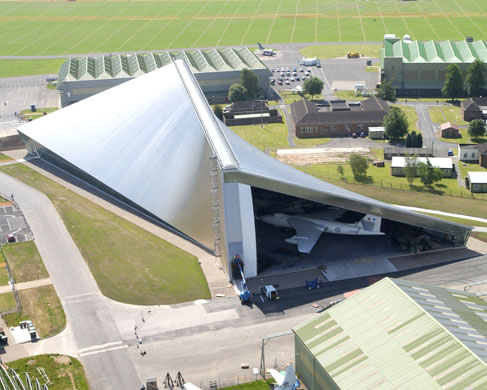This aerial color photograph captures a bustling airport complex. At the center is a large, shiny silver airplane hangar with a distinct, highly sloped roof on the right side. Inside the hangar, a sleek, modern white jet with gray wings and markings is prominently visible. Surrounding the hangar are various paved roadways and runways. The scene is bright and filled with daylight, showcasing several smaller buildings in the vicinity, including a notable red brick structure with a black roof. Two larger rectangular buildings with greenish roofs frame a busy parking lot filled with numerous vehicles. Beyond the built environment, expansive green grassy areas add vibrant contrast to the bustling aviation infrastructure below.